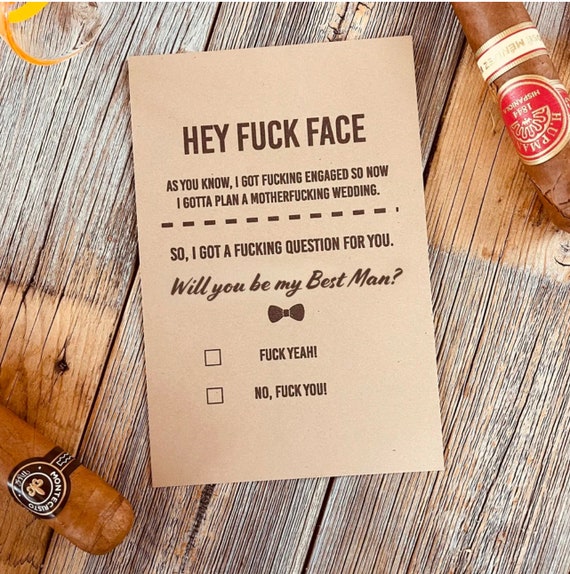The vertically rectangular, full-color photograph features a light brown paper card with dark brown text resting on a weathered, cracked wooden table. The background, likely outdoors, lacks a border and noticeably displays the rustic character of the wood. Dominating the upper right-hand corner is a cigar with a red and gold label, while the lower left-hand corner hosts another cigar with a brown and white label, each partially off-screen. The card itself starts with a bold, attention-grabbing "Hey fuckface" at the top. Below, in slightly smaller text, it reads, "As you know, I got fucking engaged, so now I gotta plan a motherfucking wedding." Further down, it asks, "So I got a motherfucking question for you, will you be my best man?" followed by humorously irreverent checkboxes: "fuck yeah" or "no fuck you." Just beneath this playful invitation, there's an illustration of a bow tie, complementing the card's brash but endearing tone.